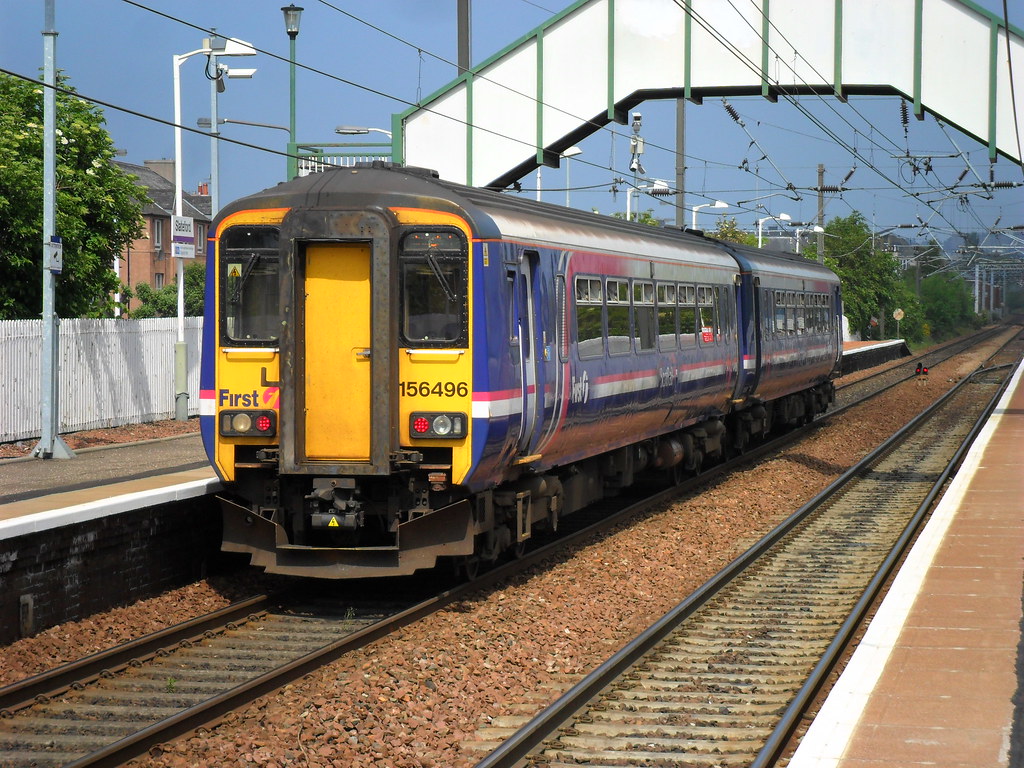This outdoor photograph captures a modern, incoming train on a clear, sunny day, set against a backdrop of a blue sky. The train, comprised of two silver cars with yellow doors and fronts, prominently displays the word "FIRST" in gray letters on the left side of the front car, along with the number "156496". The train is traveling on the left set of two parallel tracks, flanked by a track without a train to the right. Between the tracks lies a bed of brown rocks and gravel.

A distinctive white, arc-shaped overhang shelters the train, while a white warning line marks the edge of the platform it approaches. Overhead, numerous electricity wires and telephone lines stretch across the scene, hinting at the possibility of an electric train. Light posts dot the landscape, though they remain unlit in the daylight.

In the distance, a brown building with a gray roof stands beyond a white fence that separates the train area from the surrounding community. The environment is accentuated with verdant elements, including green trees and a walkway with green and white lines crossing above the tracks. Red and white stripes add vibrant accents to the train’s sides, contributing to the overall colorful and dynamic composition of yellow, purple, red, white, green, gray, brown, and black hues.